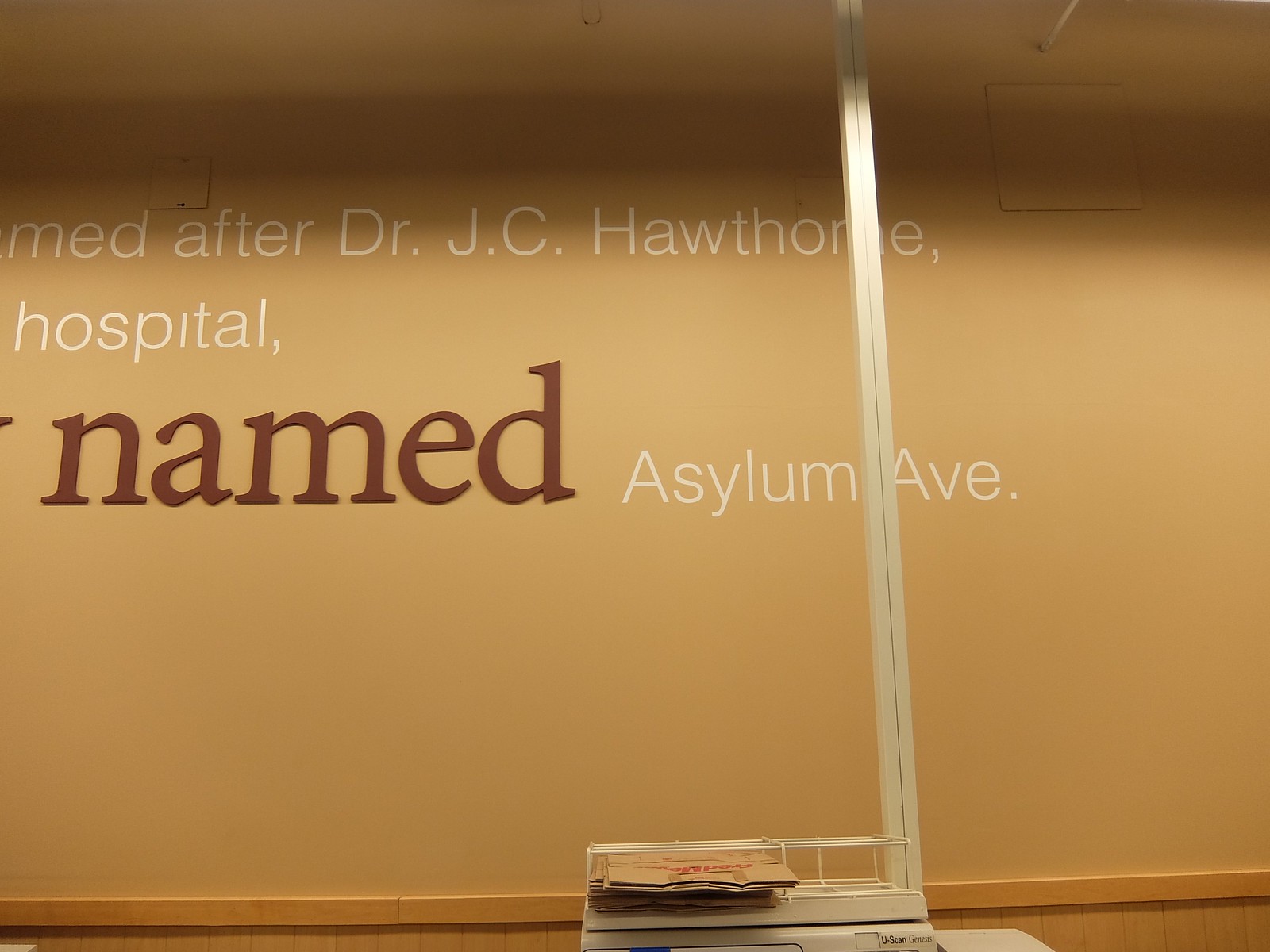The image depicts a light brown, faux wood wall that appears to be part of a hospital. A white vertical divider, possibly aluminum, runs roughly two-thirds of the way from the left side of the image. Mounted on the wall is a white wire basket located toward the lower center of the picture, containing what appear to be paper bags. Prominently displayed on the wall is a partially obscured phrase: "M.E.D. after Dr. J.C. Hawthorne," followed by "hospital," "named" in large bold red letters, and "asylum ab" in white letters, signifying it as an establishment named Asylum Avenue. The last word appears to be cut off, making the full text unclear. The overall dimensions of the image suggest it is about 20% wider than it is tall.